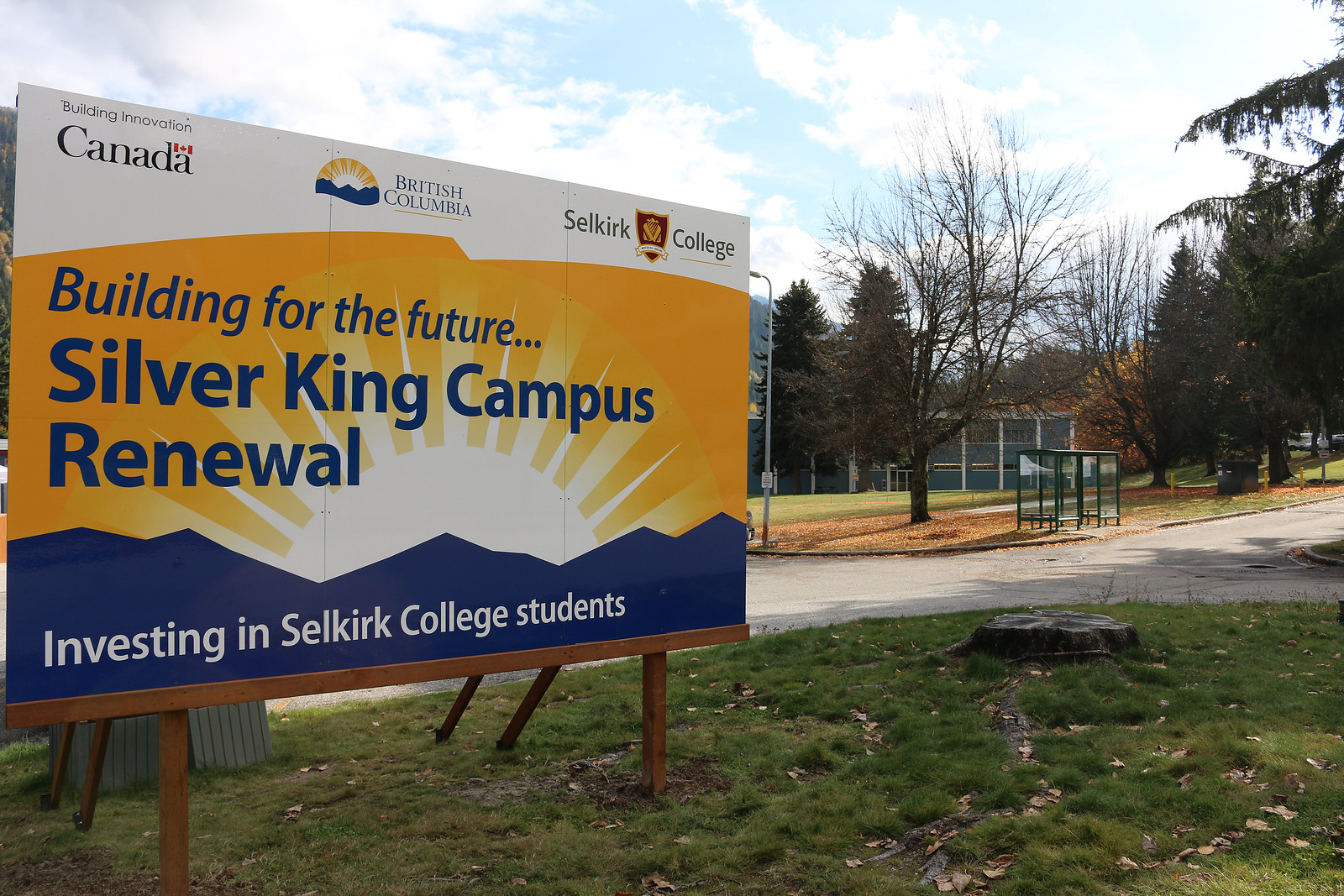In this detailed outdoor scene, we find ourselves on a college campus during the middle of the day. The foreground features a grassy field with a prominent tree stump, bordered by a roadway. Across the road lies another grassy area, which hosts a bus stop, and is surrounded by numerous trees that reach into the sky, giving a lush backdrop to the image. On the left side of the image stands a large, eye-catching billboard. The billboard reads "Building Innovation Canada, British Columbia, Selkirk College" at the top, and features the college's shield in the middle. Below the shield, in blue text against a backdrop of a sunset and rising sun, it says "Building for the Future, Silver King Campus Renewal." At the very bottom, in white text overlaying an image of mountains, it states "Investing in Selkirk College Students." The colors visible in this scene range from various shades of green and brown in the grassy fields and tree stump, to the dark blue, light blue, orange, red, maroon, gray, and black featured on the billboard and around the campus.